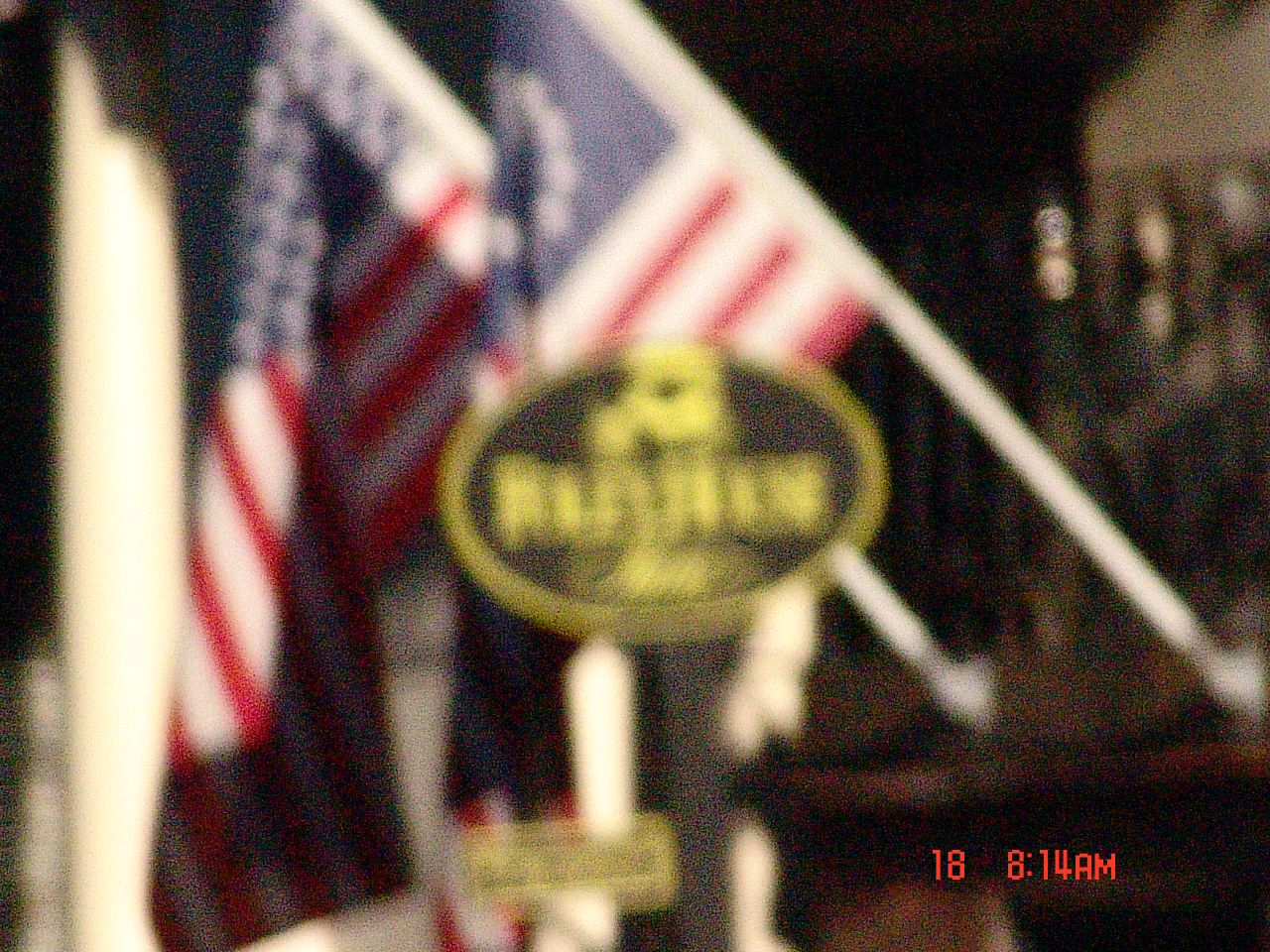This grainy image features two prominent flags displayed against a backdrop. The first is a typical American flag, with a blue field of stars positioned in the top left corner, accompanied by alternating red and white stripes. This flag is partially obscured by another flag in the foreground, which appears to be an earlier version of the American flag. This older flag bears a blue field in the top left corner, adorned with a ring of white stars, likely representing the original 13 states of the union. Both flags are mounted on white flagpoles, hanging at an angle from a dark-colored bracket, possibly wood.

In the foreground, a brown and yellow sign is visible, although the text on the sign is not legible due to the image's graininess. At the bottom right corner of the image, the numbers "18" and "814AM" are printed in red, possibly indicating a timestamp or some form of labeling. The overall setting suggests a historical or patriotic display, with the weathered appearance of the image adding a nostalgic touch.